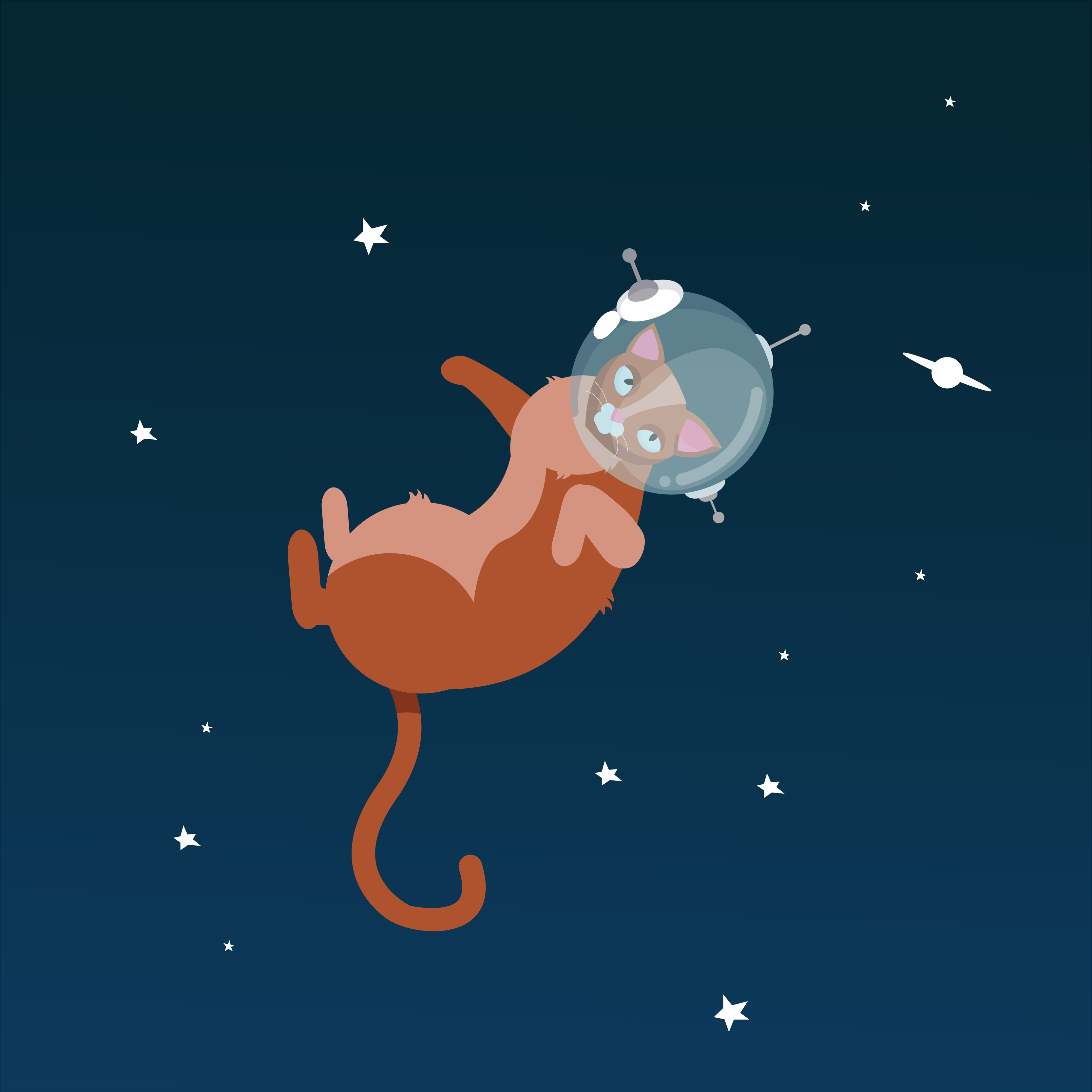The image is a detailed cartoon illustration of an astronaut cat floating in a space setting. The background is a solid dark navy blue, representing the nighttime sky, which is dotted with small white stars of varying sizes. On the upper right side of the image is a white planet with a distinctive ring around it, most likely depicting Saturn.

In the center of the illustration, the cat is floating with its belly facing the upper left corner and its long tail curling upward like a hook. The cat is primarily orange and pink in color, with rich brown fur on its back and tail, and a lighter brown-pinkish tint on its stomach area and one of its arms. The cat's facial features include large white eyes with tiny black pupils, a white nose, and a stripe running down the middle of its head. Its ears are triangular and vividly pink inside.

The cat is wearing a transparent, circular helmet with a glassy window that reveals its head and three antennae sticking out—one gray antenna on the top and two others, including a white one with a gray bar on the left side. The cat's overall position and expression give the impression that it is looking directly at the viewer, adding a sense of interaction to the animated scene. 

This whimsical and detailed science fiction illustration evokes a sense of floating and exploration, capturing the playful and curious spirit of an astronaut cat amid the stars and planets.